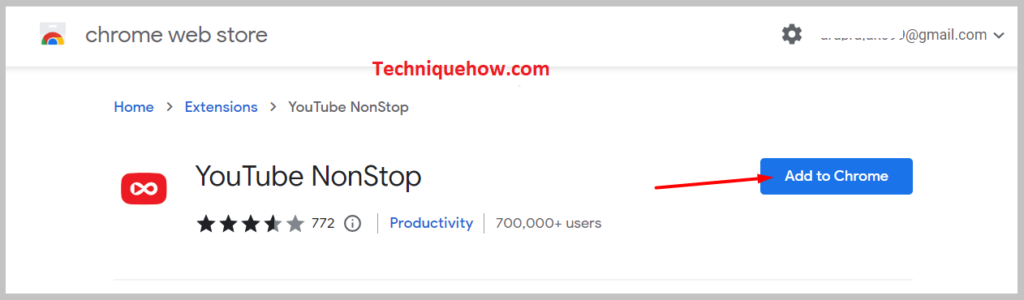In the Chrome Web Store, a user is browsing an extension titled "YouTube Non-Stop." The extension is visually represented by a red button featuring a white infinity symbol laid sideways, reminiscent of the YouTube logo integrated with an infinite playback concept. The extension holds an average rating of approximately 3.5 out of 5 stars, derived from 772 reviews, and is categorized under productivity, boasting over 700,000 users. The user has added a red arrow pointing towards the blue "Add to Chrome" button, indicating the option to install the extension. Their Gmail account is visible but anonymized, showing only "@gmail.com" due to a white overlay. A watermark reading "TechniqueHow.com" is placed on the image. The layout of the Web Store page is simple and clean, predominantly featuring a white background with black text and occasional blue hyperlinks. The Chrome Web Store icon is displayed at the top-left corner, symbolized by a colorful Google circle on a shopping bag.